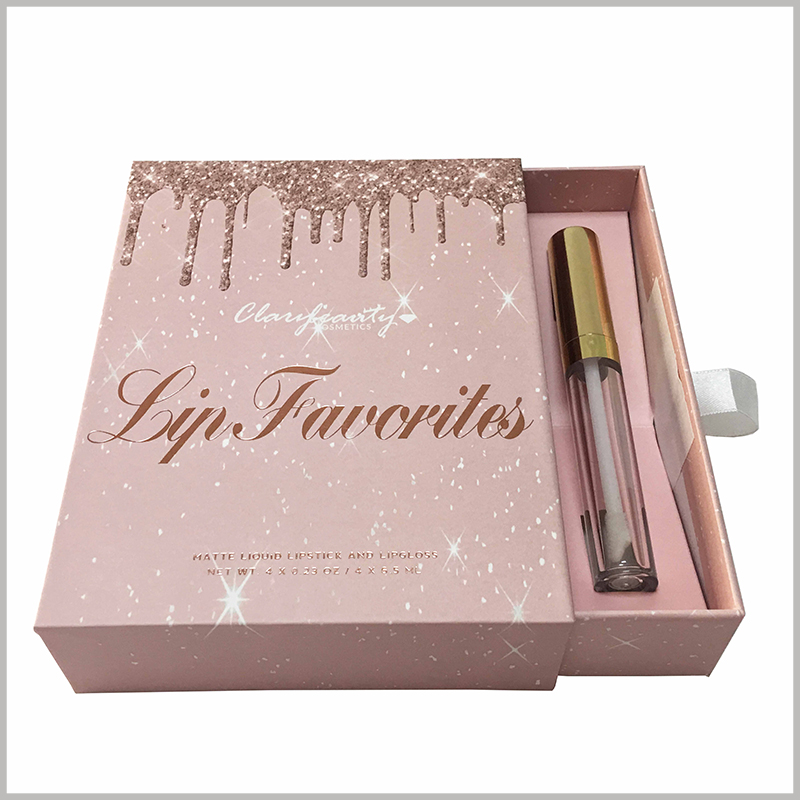The image features a pretty and charming lip product set within a pale pink box, highlighted by a thin violet borderline on a white background. The box, which opens from the right-hand side with a little white ribbon pull-out, contains four lip favorites, including matte liquid lipsticks and lip glosses. Each product has a glass bottle with a clear base and a gold cap, revealing a small applicator brush inside. The box is adorned with glittery paint dripping from the top and dotted with little shiny white stars, closely resembling a strawberry cupcake with icing. In large cursive brownish lettering, it reads "Lip Favorites" at the center, with "Claire of Ferti Cosmetics" elegantly written above in smaller cursive. At the bottom of the box, in small gold font, it specifies "Matte Liquid Lipstick and Lip Gloss" with the net weight labeled as 4 x 0.23 ounces, or 4 x 5.5 mils.